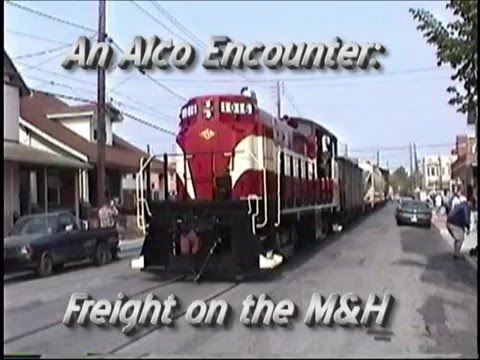A square poster with a clear blue sky background features a bustling small town scene. Multiple power lines stretch across the top left side of the image, attached to poles near a row of houses. An older-style dark gray or black truck is parked in front of one of these houses, with a person leaning on the truck bed, scratching their head. Dominating the scene, a red and white train marked with the number 1016 is running down the asphalt road that cuts through the center. The train has a rail at the front, which adds to its vintage appearance. To the right of the train, a dark-colored car is parked on the opposite side of the street. The overall setting suggests an era reminiscent of the late 80s or early 90s. In large gray text above the train, the poster reads "an ALCO encounter," while the phrase "freight on the M and H" is printed below, hinting at the freight train's function of transporting goods between towns.